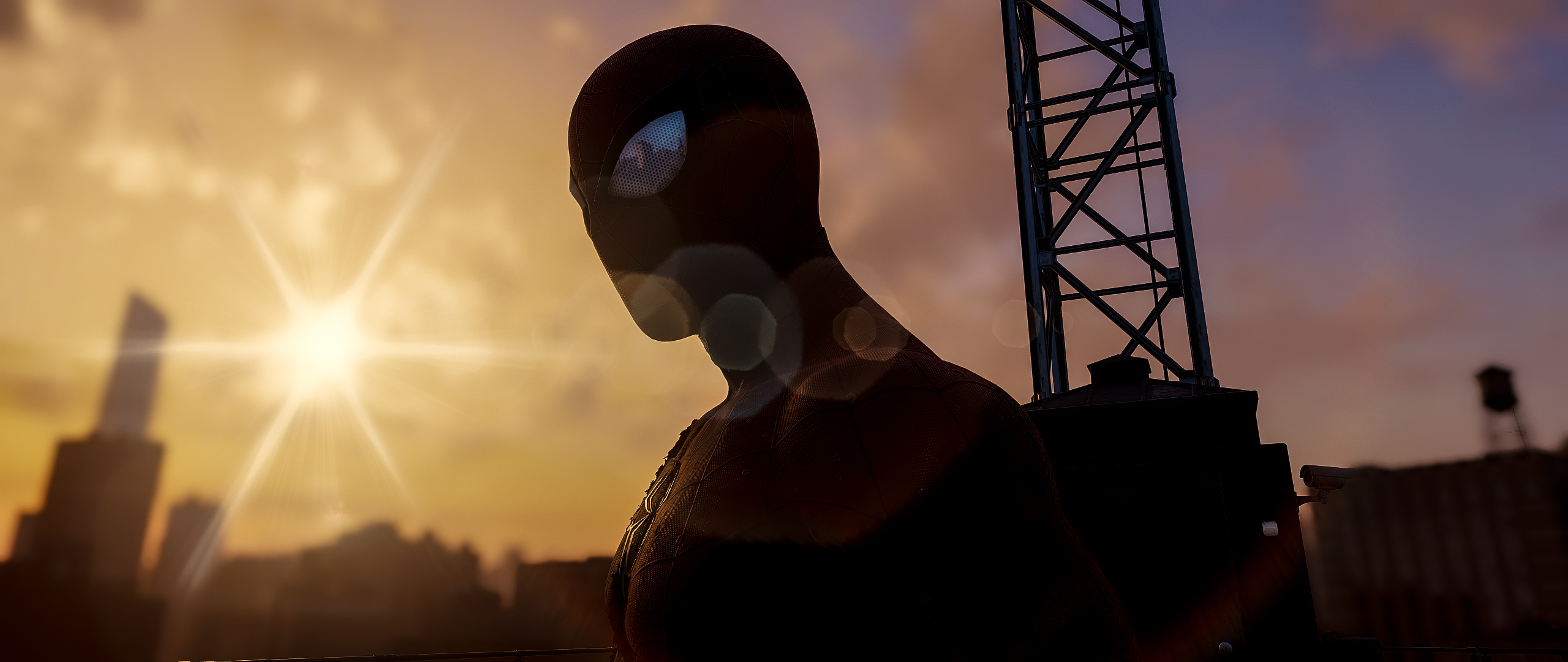A blurry screenshot from a movie scene captures a side profile of Spider-Man against a stunning sunset backdrop. Spider-Man, clad in a full black bodysuit with silver, almond-shaped, reflective eyes, stands silhouetted against the low sun, which casts a brilliant starburst of bright yellow and white light across the sky. The background features a New York city skyline filled with building silhouettes and a prominent tower to Spider-Man's right. On the horizon, an elevated water tank and a metal-post tower are also visible beneath a sky transitioning from blue to pink with wispy clouds. The sun's glow and the silhouettes combine to create a stark contrast, highlighting Spider-Man's dark figure and the silvery detail of his eye.